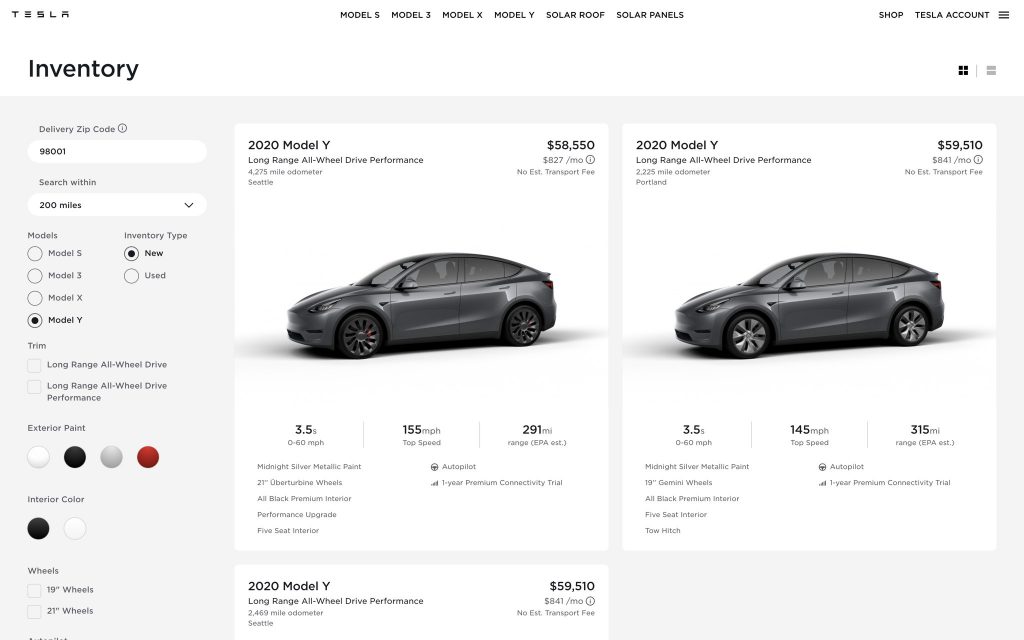This image is a detailed screenshot of the Tesla website, which primarily features a clean, white background. At the top left corner of the screen, the word "Tesla" is prominently displayed. Centrally aligned along the top are links to different Tesla products: "Model S," "Model 3," "Model X," "Model Y," "Solar Roof," and "Solar Panels." On the far right, you find navigation options including "Shop," "Tesla Account," and "Inventory."

Towards the left-hand side of the screen, the word "Inventory" is highlighted in large black letters. Below this heading, the website layout showcases two Tesla cars in a typical e-commerce fashion. The first featured vehicle is a 2020 Model Y Long Range All-Wheel Drive (AWD) Performance, priced at $58,550, or available for financing at $827 per month. Key specifications such as "Long Range" and "All-Wheel Drive Performance" are listed beneath the vehicle.

Adjacent to the first, the second car displayed is also a 2020 Model Y Long Range AWD Performance, but this model retails for $59,510. A third vehicle option is mentioned below, though its image is not visible in this screenshot.

In the left-hand margin next to the car images, users can find additional tools to refine their search. These options include entering a delivery zip code, defining a search radius in miles, selecting different car models, specifying whether the car is new or used, and choosing preferences for exterior paint, interior color, and wheel dimensions.